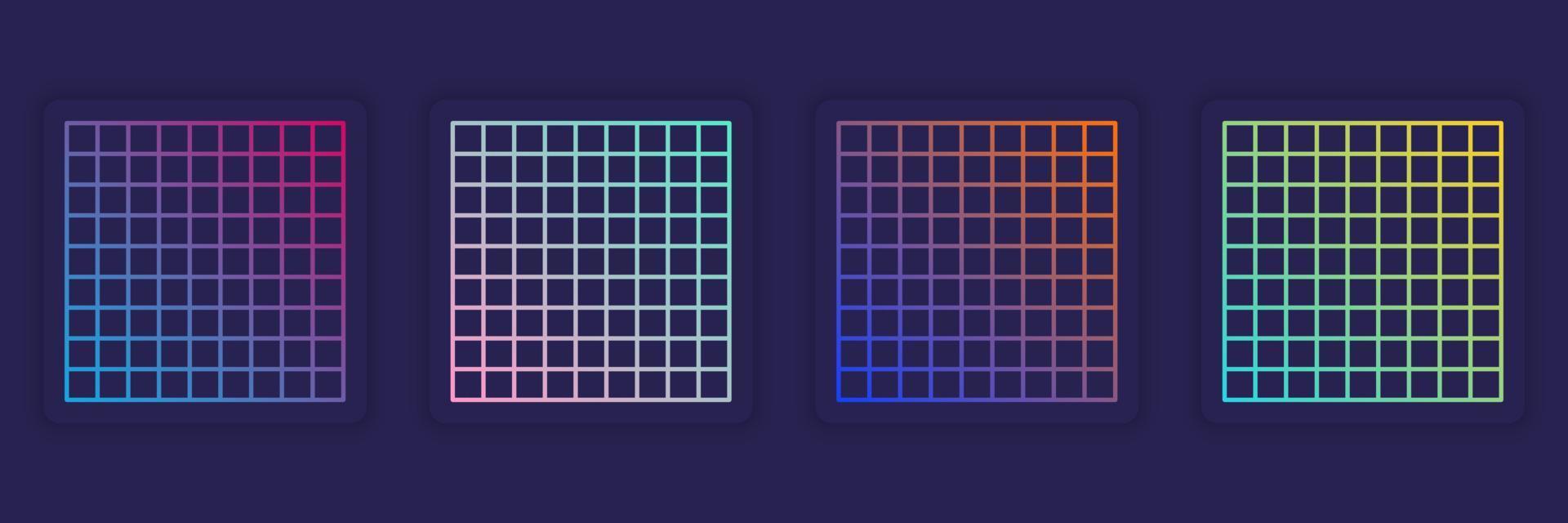This image features a landscape-oriented digital artwork with a deep purple or nearly black background. The main focus is a series of four large, evenly spaced squares arranged horizontally across the center. Each large square is subdivided into an 9x9 grid of smaller squares, making a total of 81 smaller squares within each large square. 

1. The first large square (starting from the left) features a gradient transition from blue in the lower left to deep pink in the upper right, passing through various shades of purple and red.
2. The second square transitions from pink in the lower left to light green in the upper right, with some white intermixed.
3. The third square begins with a deep blue in the lower left, moves through lavender and purple shades, and ends in a rusty orange at the upper right.
4. The fourth square starts with an aqua color in the lower left and transitions through greens, finally fading into various shades of yellow in the upper right.

There are no text, numbers, or other elements present in the image, lending it a minimalist appearance that could suggest either abstract art or a scientific visualization.